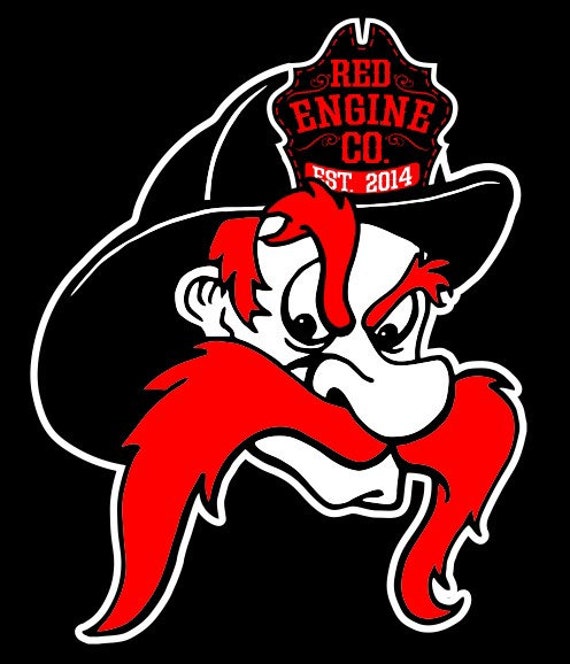The image features an advertisement poster or logo set against a completely black background, focusing solely on the illustrated head of a cartoonish fireman. This character has a stark white face, a very big nose, and a sharp chin, all contributing to his mean and angry facial expression. His most striking features include his bushy, flame-red mustache and thick, expressive eyebrows, both outlined with big, thick black lines, and a matching red hair. He is depicted wearing a black fireman's hat with white outlines. Prominently displayed on the front of the hat is a shield emblem with red text that reads "Red Engine CO." in separate lines and a red banner below it that states "EST. 2014." The character's exaggerated, animated style makes the features, particularly the long, handlebar mustache, stand out vividly against the dark background, emphasizing his fierce demeanor.